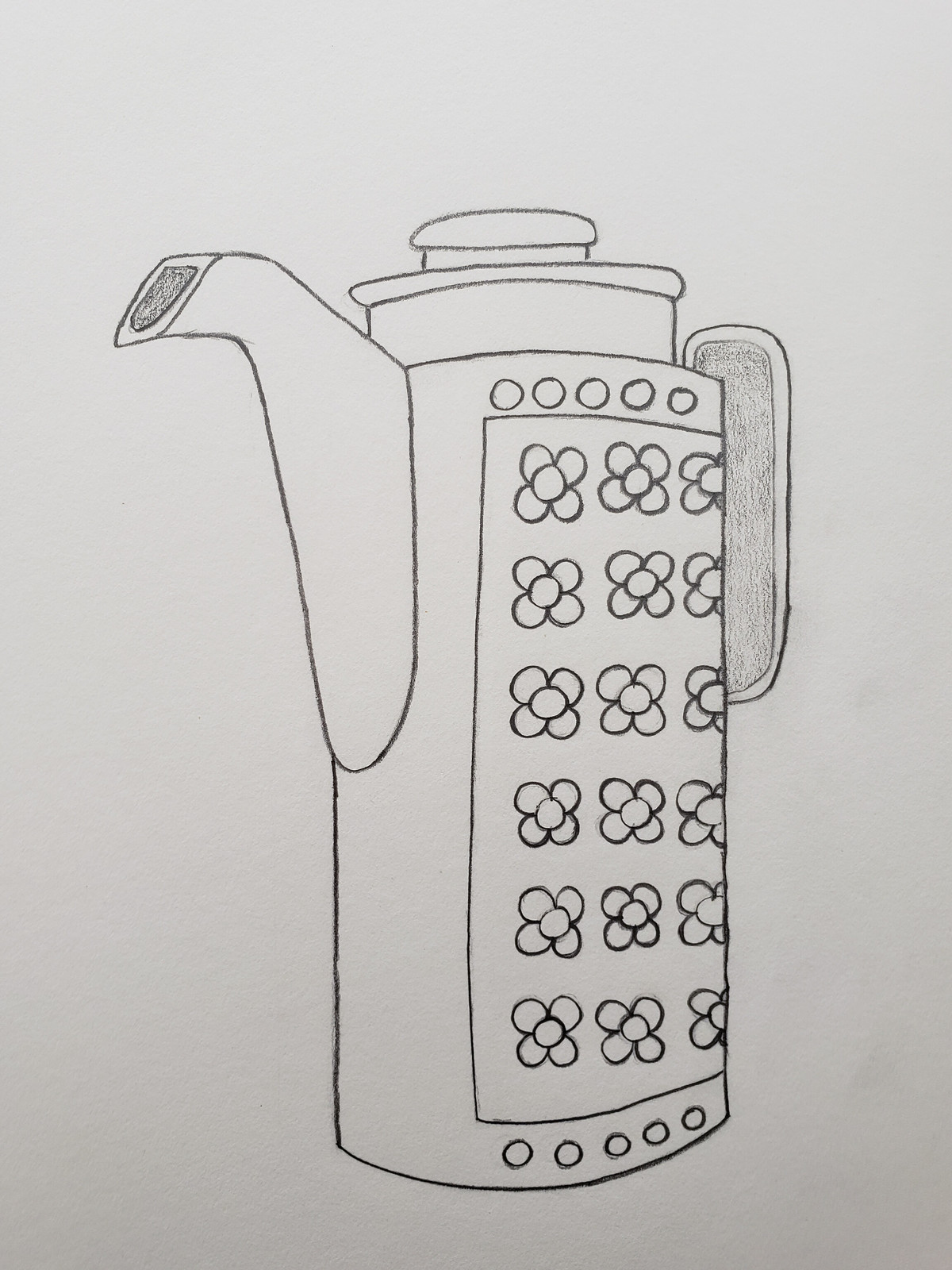This detailed pencil drawing depicts an unusually tall teapot that resembles a pitcher in size and shape. Rendered in dark pencil on a white backdrop, the teapot features an elongated body commonly associated with pitchers used for serving water or juice. The teapot is adorned with a tall lid and a tea spout, adding to its unusual appearance. Decorative elements include a pattern of flowers intricately drawn in a rectangular section near the center, organized in a grid-like pattern. Additionally, there are five detailed circles placed at the top and bottom of the teapot, enhancing its whimsical design. A handle is situated on the right, extending gracefully, while the spout protrudes to the left. The artwork relies solely on shading techniques, showcasing a range of pencil shades to emphasize texture and depth.